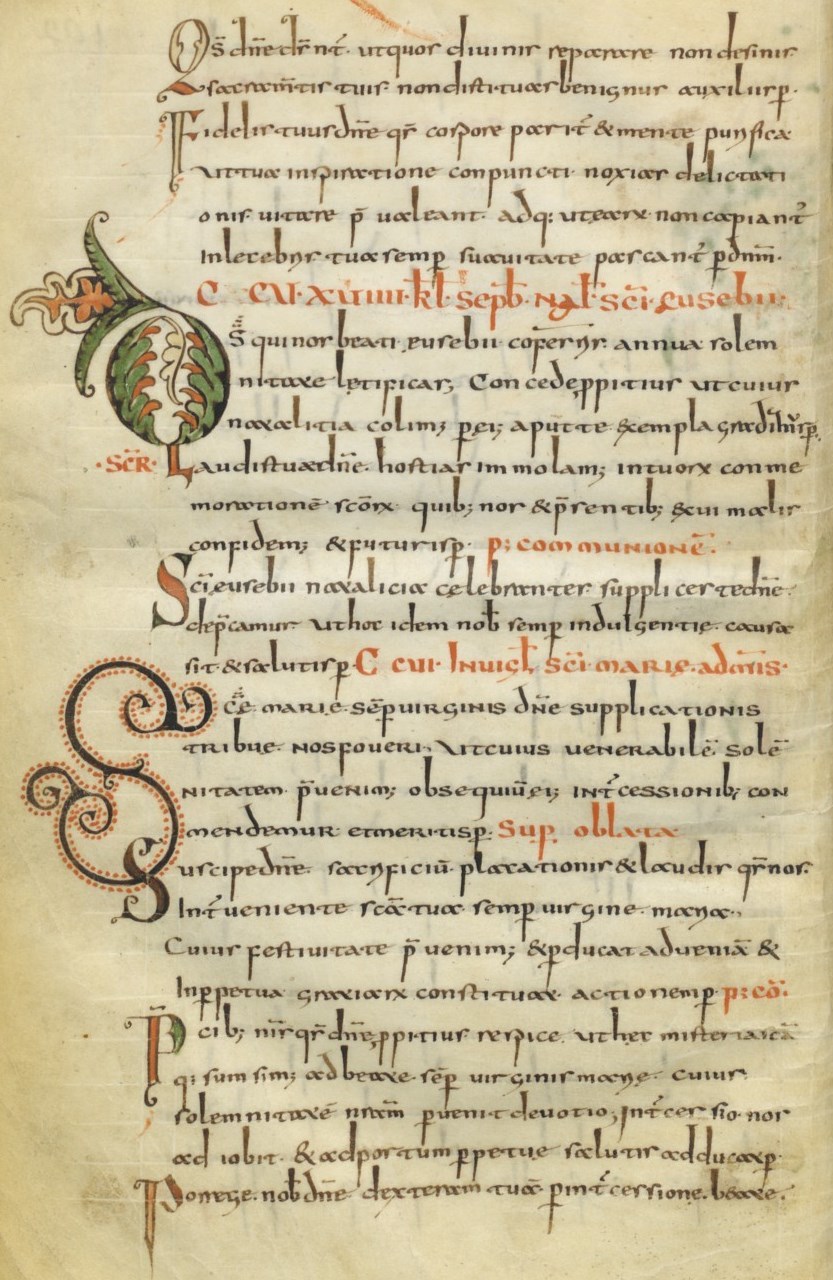This image, a color photograph in portrait orientation, features an antique printed page with handwritten typography and elaborate decorative initials. The aged beige parchment, resembling cream-colored stationery, contains text in a foreign language, predominantly in black ink, interspersed with a few words in orange-red. The text spans approximately 25 lines, neatly scripted in an ornate font. Prominently, the top left showcases a large decorative 'O', artistically rendered with leafy flourishes and flowers. Further down, a meticulously crafted 'S' is adorned with intricate swirls and red dots. Additional decorative initials, including 'Q', 'T', 'P', and another 'S', contribute to the page's sophisticated aesthetic. The left side of the page, if viewed while writing, features various small, scripted illustrations, completing the vintage, representational realism of this hand-printed document.